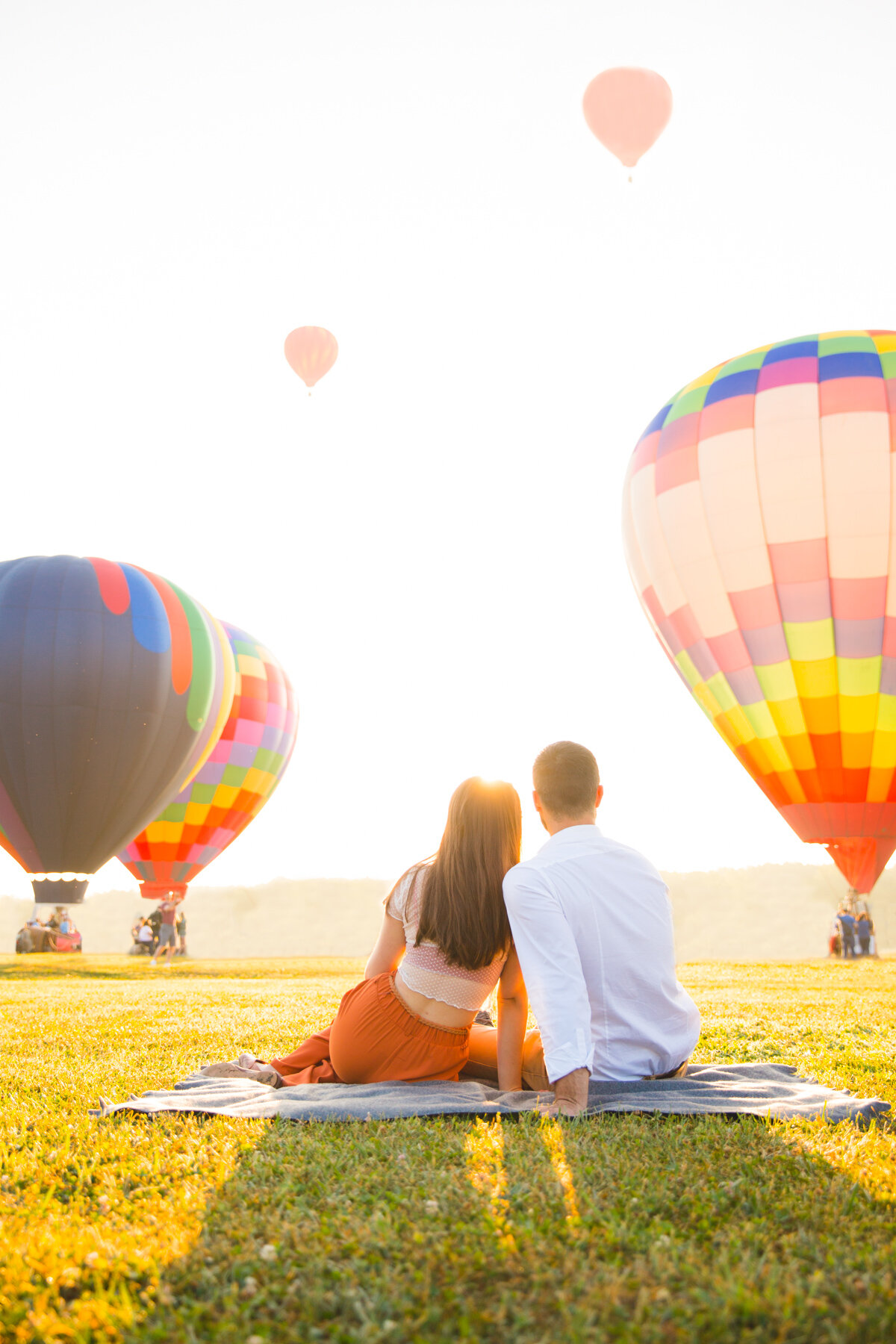In this vibrant and detailed color photograph taken from ground level, a couple is seated on a gray picnic blanket on a lush, green grass plane, their backs facing the camera. The man, positioned to the right, is wearing a long-sleeved white dress shirt and has short hair. He is seated shoulder-to-shoulder with a woman on his left, who is dressed in a short-sleeved, tight-fitting white top and loose orange pants, her long brunette hair resting against his shoulder. They are both gazing out at the scene before them. The day is sunny yet slightly hazy, likely due to lens flare, imparting a dreamy quality to the image. In the background, several groups of people, possibly families, are seen preparing hot air balloons. Three colorful balloons, adorned in shades of red, yellow, purple, and white, are on the ground, while two red balloons ascend into the sky. The overall atmosphere is serene and filled with the anticipation and wonder of hot air ballooning.